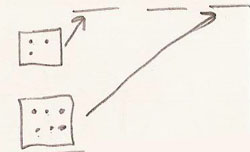Title: Minimalist Graphite Diagram with Geometric Annotations

Caption: This intricate yet cryptic graphite sketch, approximately the size of an index card, is crafted with precise, albeit rough, geometric forms. The upper right corner features three spaced dashes, reminiscent of incomplete hangman marks. On the left side, an imperfectly drawn box sits near the top, filled with three dots arranged like a domino: one in the upper left, one in the bottom left, and one in the upper right. An upward-pointing arrow extends from this box to the first dash. Below this, another irregular box is populated with six dots, arranged in two rows of three. A lengthy line stretches from this second box to the upper right, linking to the third dash. Despite the meticulous detailing of lines, dots, and arrows, the sketch's purpose and message remain enigmatic, leaving its interpretation open to the viewer’s imagination.